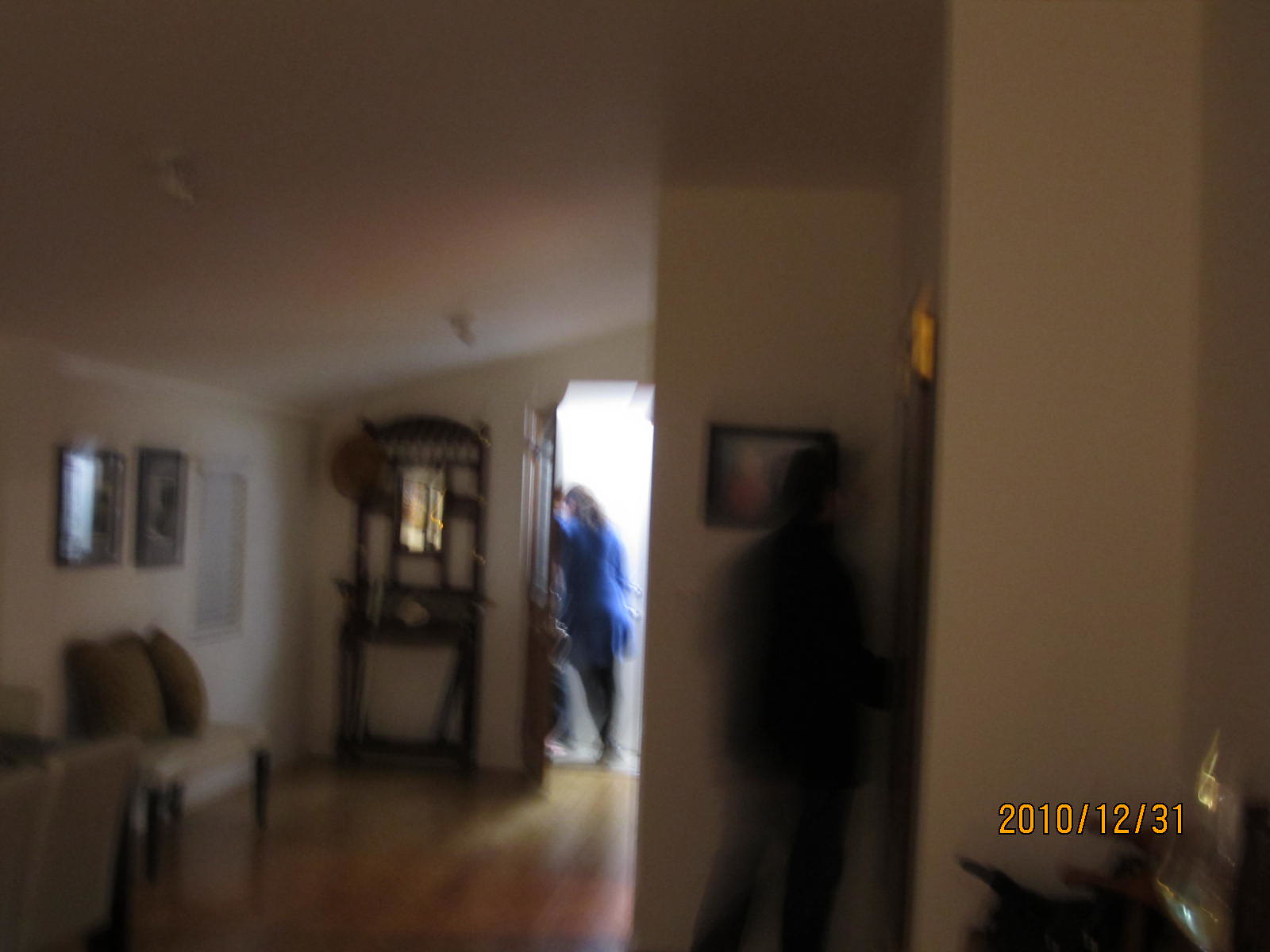Caption: 

Photograph dated December 31, 2010, capturing a New Year's Eve gathering in a uniquely shaped room. The room features a sloping roofline descending to the left and is accessed through a front door visible in the image. In the background, one individual in dark clothing, possibly jeans, appears blurry as they interact with a protruding wall or closet door adorned with a picture. The wooden floor adds warmth to the scene.

The foreground centers on a person dressed in a blue top and a skirt or dress with black leggings, engaged in conversation with another individual at the open doorway. Bright light streaming through the doorway contrasts with the otherwise dim and slightly blurred interior. To the left, a fancy coat rack stands beside the door, and a few paintings decorate the wall. The room is sparsely furnished with a few chairs, none of which appear particularly comfortable.